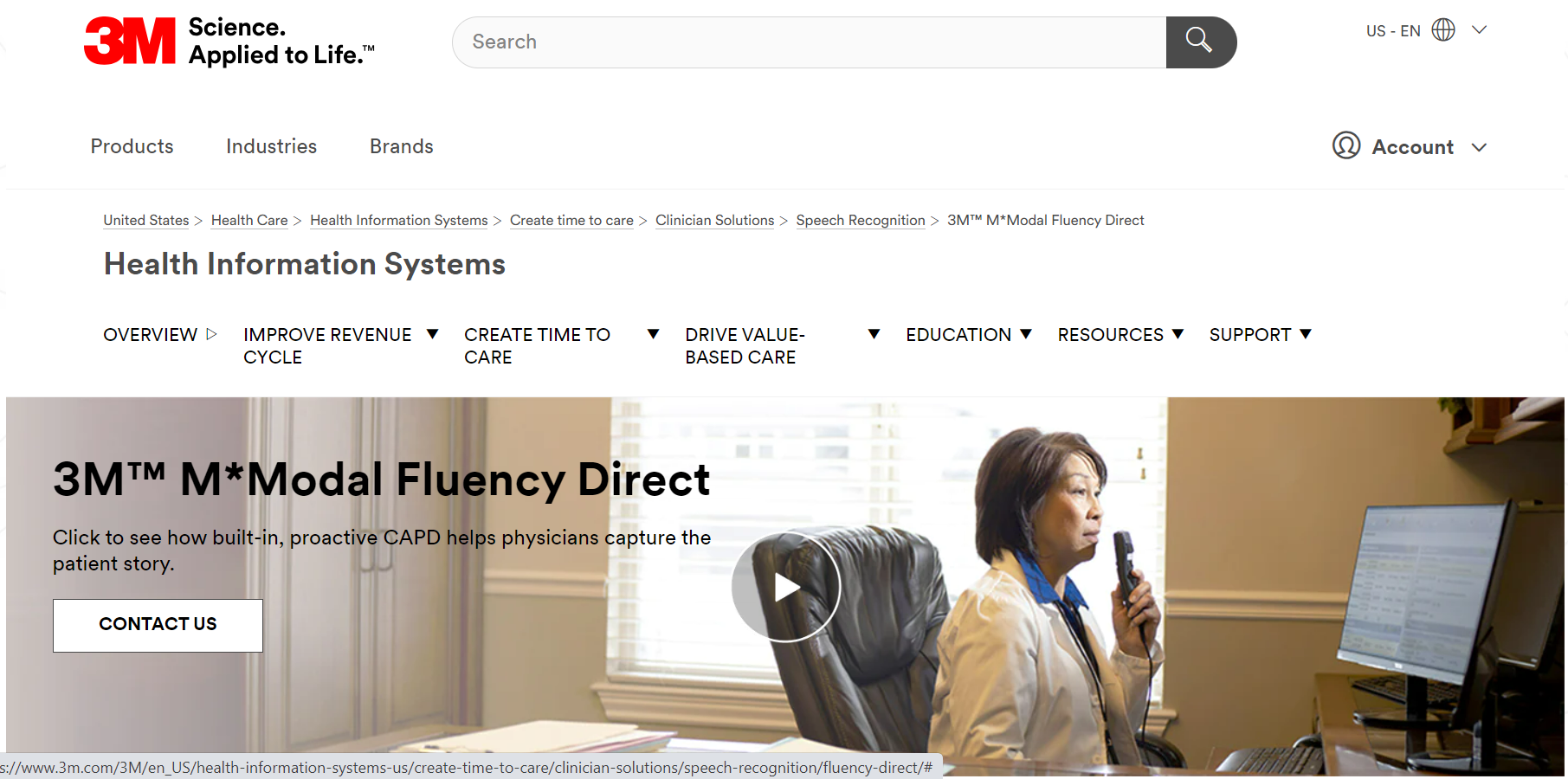The image is a screenshot taken from a 3M website. In the top left-hand corner, the bold red "3M" logo is prominently displayed, accompanied by the tagline "Science Applied to Life" in black font. Adjacent to the tagline, on the right side, is a blank search bar. 

The central part of the page features various categories listed horizontally, including "Overview," "Improve Revenue Cycle," "Create Time to Care," "Drive Value-Based Care," "Education," "Resources," and "Support."

At the bottom of the image, there is a small video preview indicated by a play button in the center. The background shows a woman seated at a desk with a computer in front of her, holding a microphone close to her mouth. To the left of this scene, the text reads "3M Modal Fluency Direct." Below this title, a description states, "Click to see how built-in, proactive CAPD helps physicians capture the patient's history."